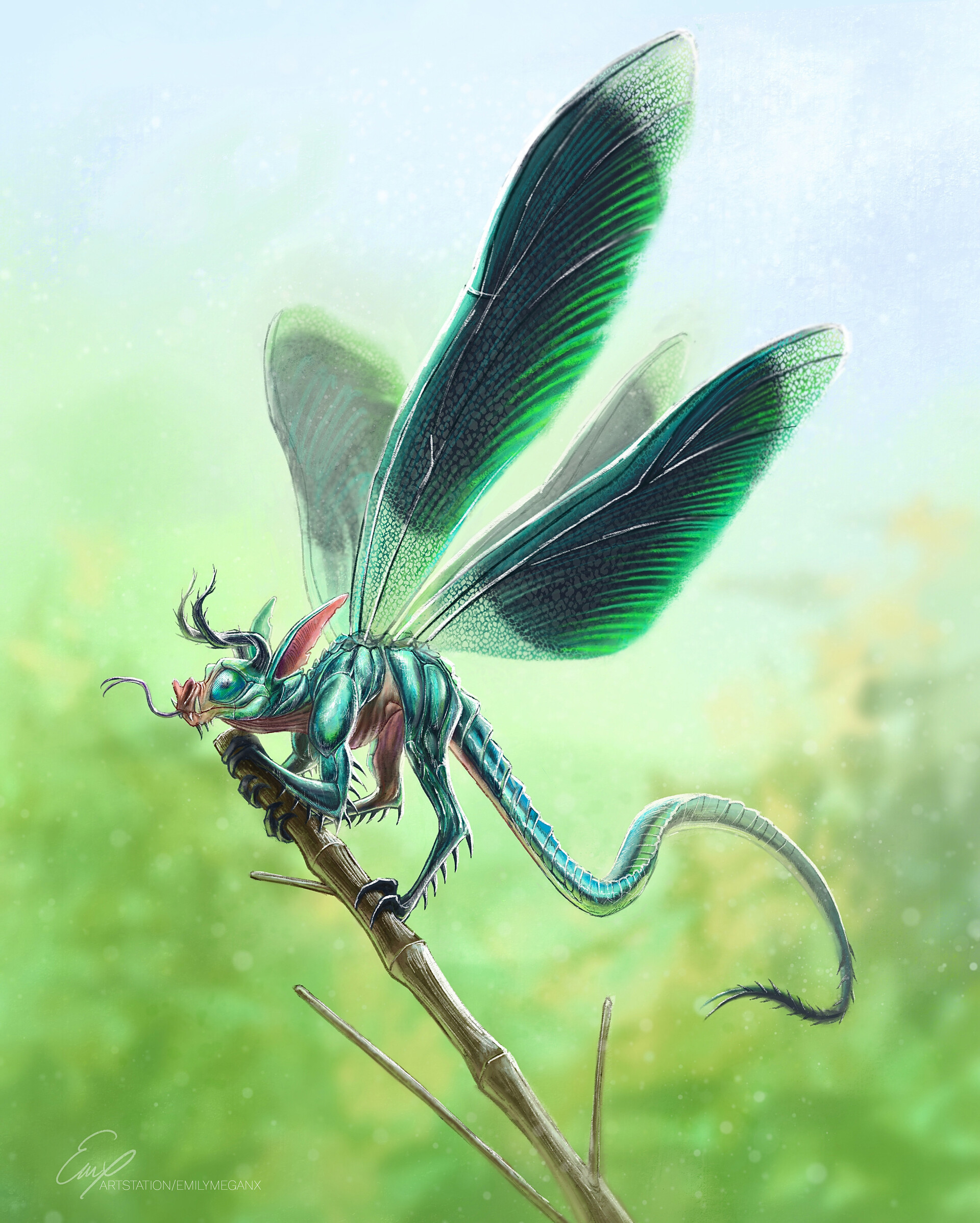This illustration captures an imaginative hybrid creature with intricate detail. The creature bears resemblance to both a dragonfly and a rat, featuring a blue, muscular body with a long, spiny tail. It is adorned with four prominent green leaves or wings, two of which are intricately detailed with a blend of black, green, and white hues. The creature's face combines characteristics of a fowl and an insect, boasting large ears, strong antennas, and whiskers, with a red tongue and underbody adding a striking contrast. Its claws are sharp and black, grasping onto a small brown twig. The background is a blurred mix of green and blue, enhancing the mysterious and otherworldly atmosphere of the scene. A cursive watermark, "Art Station Emily Megan X," is faintly visible in the bottom left corner.